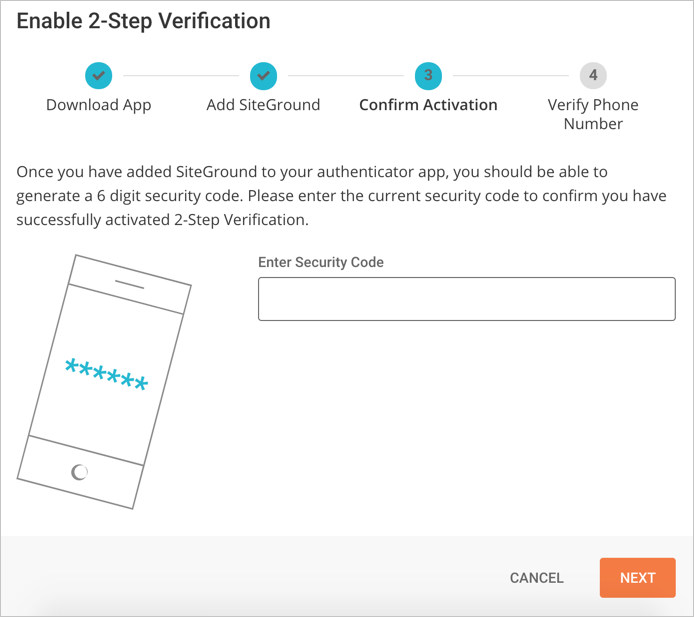A detailed visual description of a screenshot depicting the two-step verification process for an unidentified website. The interface is predominantly black and white, with a clean layout. At the top, a progress bar divided into numbered steps guides the user through the verification procedure. 

**Step 1**: "Download the app" - Marked with a blue checkmark indicating completion.
**Step 2**: "Add SiteGuard" - Also marked with a blue checkmark, showing it has been completed.
**Step 3**: "Confirm Activation" - Highlighted as the current step, lacking a blue checkmark as it's still in progress.

Following this, the next step, **Step 4**: "Verify Phone Number," is outlined as the subsequent task.

Instructional text just below these steps reads: "Once you have added SiteGuard to your Authenticator app, you should be able to generate a six-digit security code. Please enter the current security code to confirm you have successfully activated two-step verification."

Beneath the instructions is a text box where users can enter a six-digit security code. Adjacent to this field, on the bottom left, is a simplistic graphic of a mobile phone, depicted as a rectangle with minimalistic details - two lines at the top and bottom representing the phone’s edges, and another line at the top symbolizing a speaker, with a centered blue asterisk placeholder for the entered code.

On the bottom right, users have the option to cancel the verification process or click "Next" to proceed after entering the security code. The page's only color, aside from black and white, comes from the blue elements, specifically the checkmarks and the step progression bubbles, adding a touch of visual clarity.